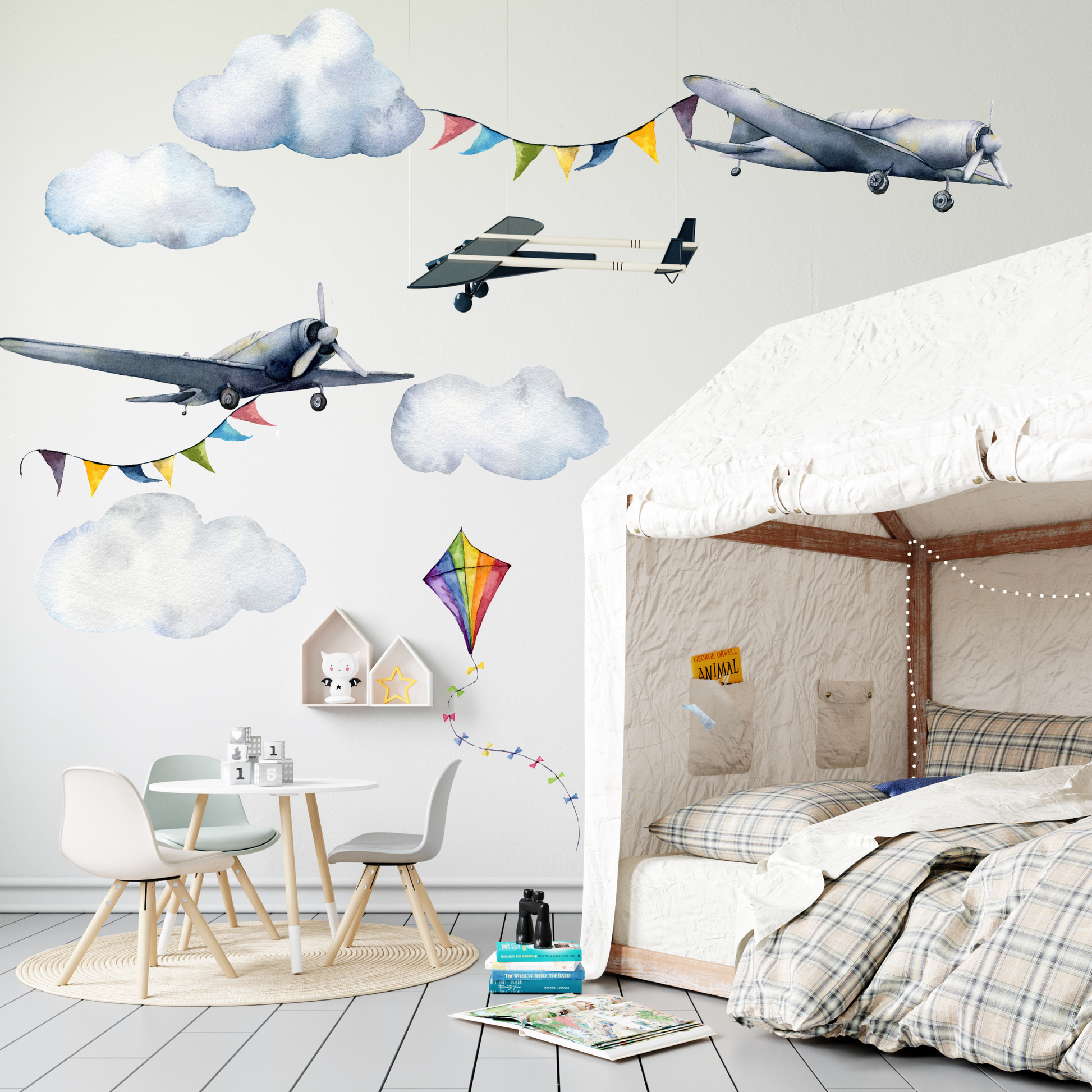The image depicts a meticulously arranged child's bedroom with a prominent aviation and flight theme. On the right side of the room is a unique bed adorned with a plaid duvet and matching pillows, including a body pillow. The bed is nestled beneath a wooden canopy structure that has a white comforter or summer quilt draped over it as an awning roof. 

The backdrop of the room features a white wall painted with fluffy, grayish clouds and several 3D airplanes complete with trailing, multicolored flags. Also painted on the wall is a vibrant rainbow kite with rainbow-colored bows on its strings, further emphasizing the flight theme.

In the foreground, there is a small, pastel-colored table set with cream, mint green, and gray chairs—each with wooden legs. On the floor, resting on the gray hardwood, are a picture book, a blue box, and a pair of black binoculars. 

Additionally, the room is furnished with two small, house-shaped white cubbies affixed to the wall, completing the whimsy and well-curated appearance of this idealistic and visually appealing child's bedroom, likely styled specifically for the photograph.